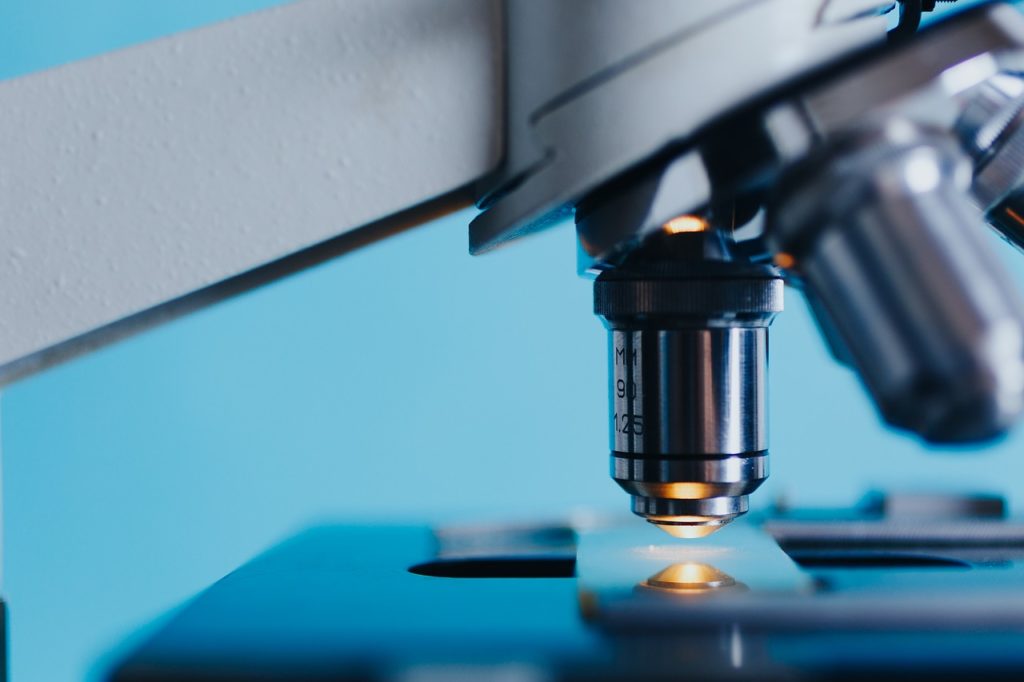This horizontally aligned rectangular picture is a close-up color photograph of a detailed section of a microscope. Dominating the upper left part of the image is a large white metal arm reaching out, with a silver cylindrical piece attached to it, which bears partially readable black print that says "MM90 1.25." This cylinder, tapering towards the bottom, appears to house a lens and has a dome-shaped light at its base, surrounded by a silver ring, shining an orange light downwards onto a rectangular metal plate. The plate is part of the larger body of the microscope, which has a shiny black surface. Off to the side, other similar silver cylindrical lenses are visible, suggesting multiple magnification options. The background is mostly light blue and blurred, emphasizing the microscope's intricate details.